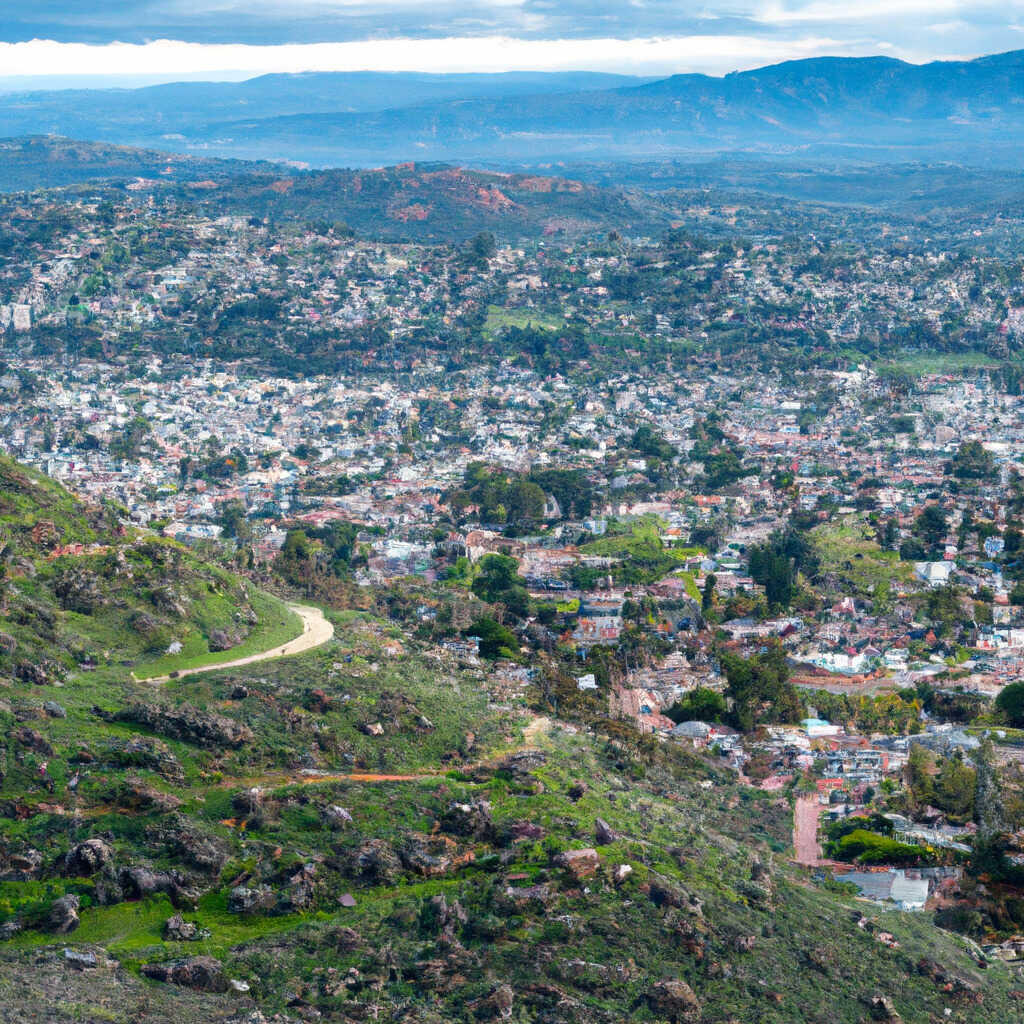In this highly detailed, panoramic image, a vast cityscape extends below a dramatic sky that transitions from gray at the top to white lower down. The city, densely packed with hundreds of buildings, lacks towering skyscrapers, suggesting a bustling yet modestly scaled urban area surrounded by countryside. Scattered among the buildings are numerous trees and bushes, adding a touch of greenery to the urban sprawl. To the left foreground, a steep, triangular green hill slopes diagonally from the middle left to the lower right corner, intersected by a small, winding yellow road. This hill gives way to a rocky expanse with patches of grass, providing a contrasting natural element to the city scene. In the background, a series of blue and brown mountain ranges rise, adding depth and beauty to the landscape. The image, rich in detail, captures the essence of a city nestled within a vibrant and varied natural setting, reminiscent of a view from a low-flying airplane.